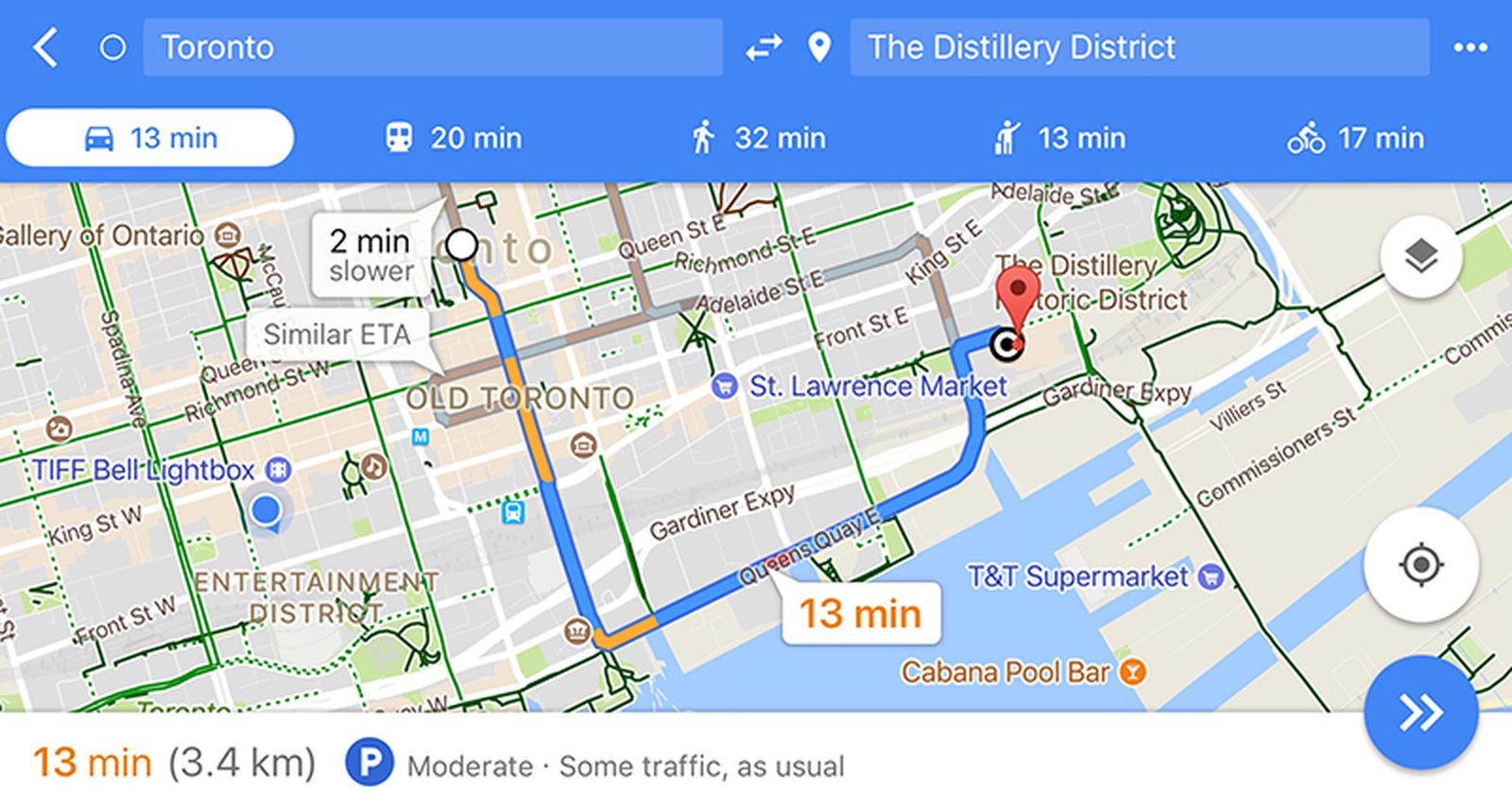The image displays a map with a search query for Toronto entered in the search bar, focusing specifically on The Distillery Historic District as the desired destination. The map header is blue and prominently features details about travel options to the district. By car, the journey is estimated at 13 minutes and covers a distance of 3.4 kilometers, with typical traffic conditions noted as moderate. Walking would take approximately 32 minutes, cycling 17 minutes, taking a bus 20 minutes, and using a taxi also about 13 minutes.

A red pin marks the location of The Distillery Historic District on the map, indicating that this is the area of interest rather than a specific restaurant. Some areas on the map are highlighted in blue, possibly indicating points of interest or significant locations.

At the bottom, a blue circle with a double white arrow is visible, suggesting an option to expand or navigate further. The top of the image features a menu icon with three dots, providing additional options for interaction. The map itself also displays surrounding areas, giving a broader context of the district’s location within Toronto.